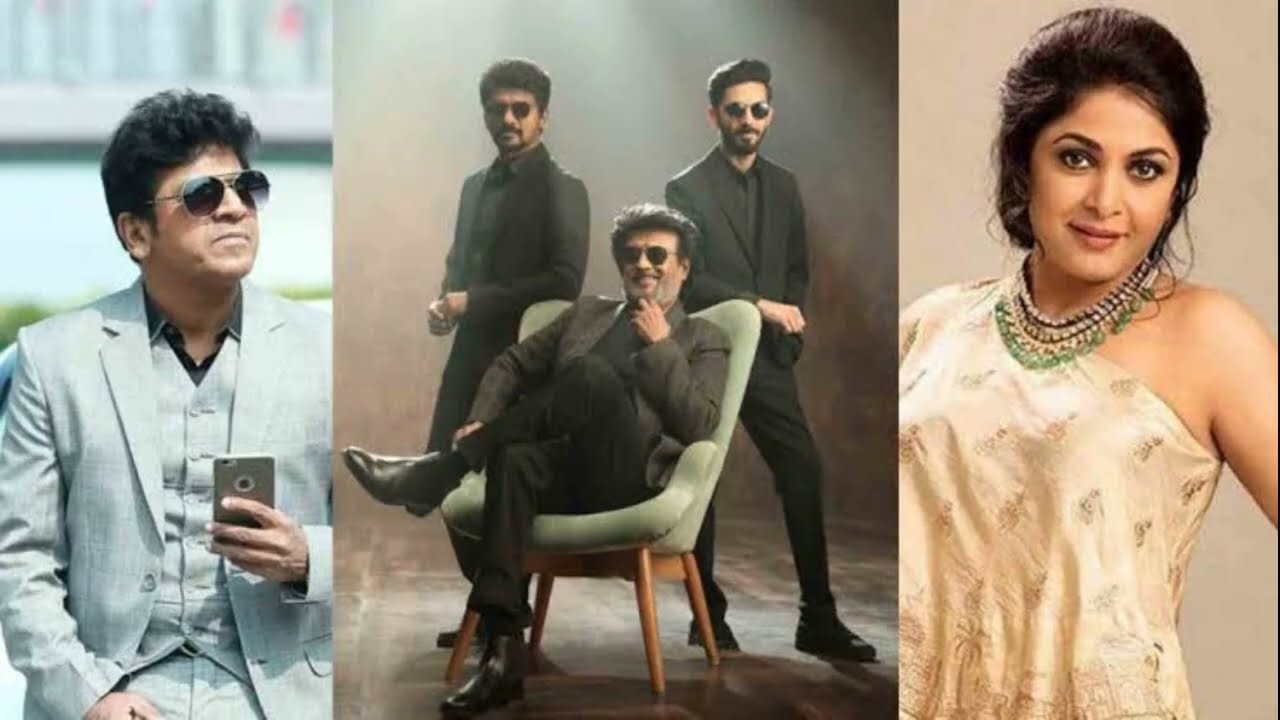The image is a triptych collage with three distinct panels. The left panel shows a man outdoors, dressed in a light gray, two-piece suit with no tie, holding a phone in his left hand. He has dark, curly hair and wears aviator sunglasses, looking slightly upward to the left. The background is out of focus but suggests a possible road or water near a building. The middle panel features three men, all in dark suits and aviator sunglasses. One man is seated in a light green, sage-colored chair with wooden legs, crossing his leg and resting his hand thoughtfully on his chin while smiling. The two other men stand behind the chair, each leaning against one corner of the backrest. The setting appears to be a tiled floor area, dimly lit. The right panel depicts a woman in a light golden, silky gown adorned with multiple necklaces, including a notable light green one among brown and beige ones. She has dark hair and a slight smile, with her left shoulder exposed and her right shoulder covered by the dress. The overall color scheme includes shades of yellow, light blue, and brown.